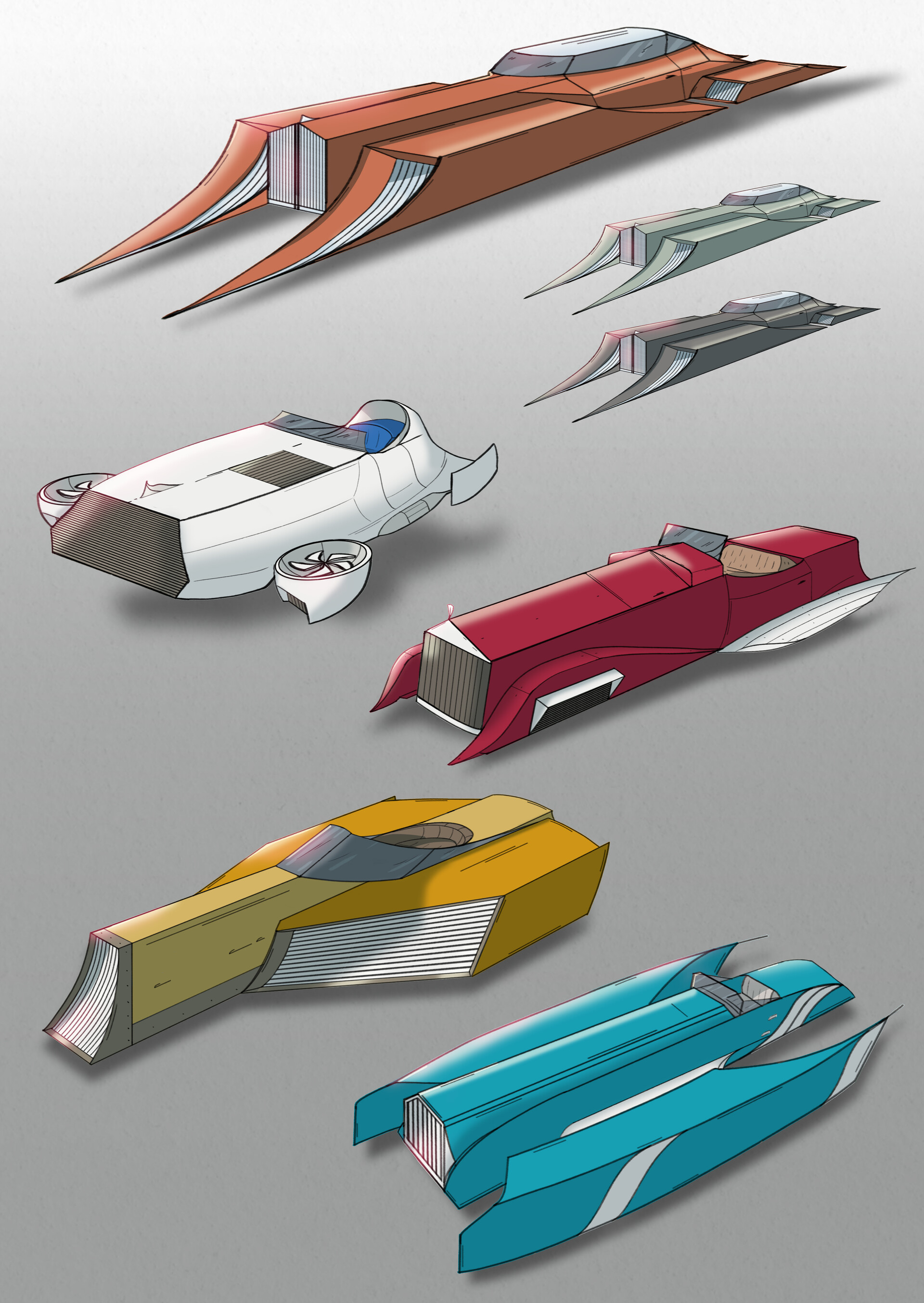The image features a detailed and colorful array of concept drawings for futuristic cars, set against a vertical gray background. Each vehicle merges modern and retro aesthetics, displaying the influence of classic Cadillacs and sports cars, but with sharper lines and more pronounced angles, giving them a sleek, avant-garde appearance. These cars appear to float slightly above the ground. At the top, an elongated, brownish-orange car resembles a large Cadillac with a long, slender body and pointed scoops in the front, maintaining a traditional Cadillac grille with a cabin situated at the back. Below it, various iterations in differing colors follow. There's a shorter, squat white vehicle resembling a personal airplane, with two propellers on each side like a drone capable of vertical takeoff. Next, a red car mirrors the Cadillac design but with slightly softer angles. Lower still, a sportier yellow car with a front scoop grill exudes a slight Star Wars vibe. At the bottom, a blue sedan with white stripes features wing-like elements. The artistic representation uses a diverse palette, including blue, yellow, red, white, brown, orange, and gray, emphasizing the futuristic ethos through both design and color scheme.